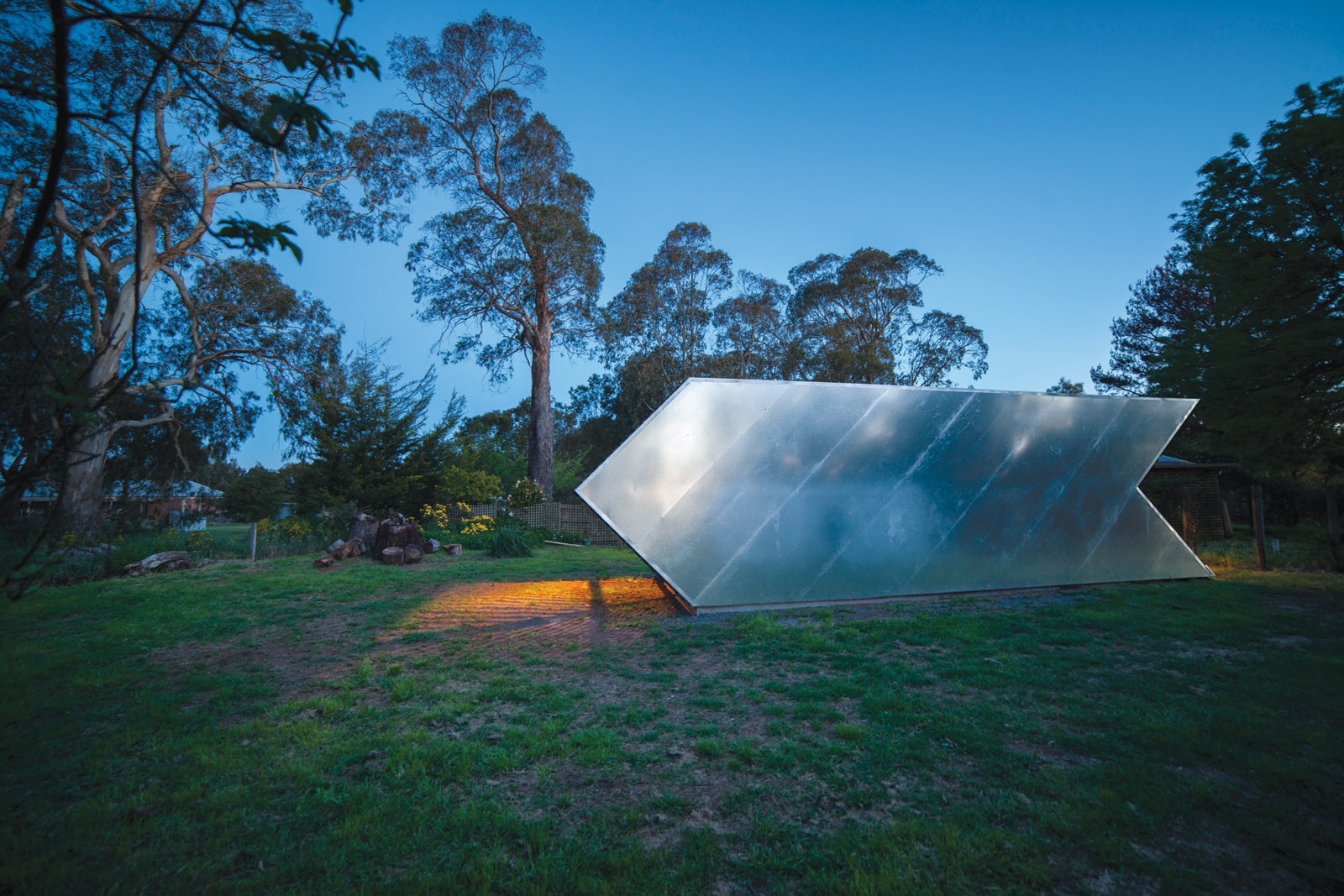The image captures a spacious backyard dominated by an expanse of green grass, though some sections in the center appear patchy and dead. Prominent in the scene is a distinctive two-paneled solar panel with a sleek, gray metallic finish, positioned as if a bench were tipped forward with its top facing the sun. Its slightly folded design evokes the look of a geometric arrow pointing left, crafted from stainless steel. 

In addition to the solar panel, the yard features a varied backdrop of large, sparse trees, some barren, others partially leaf-covered, accentuating the geography's resemblance to an Australian landscape. The clear, cloudless blue sky further enhances the scene's open, airy feel.

Towards the corner of the image, some flower beds and rocks are visible, possibly accompanied by a shed. Illuminating the scene, presumably artificial lights shine on the back end of the solar panel, suggesting evening or twilight as the time of day. The structure's reflections and the light emanating from it add a touch of modern artistry to the rustic outdoor setting.